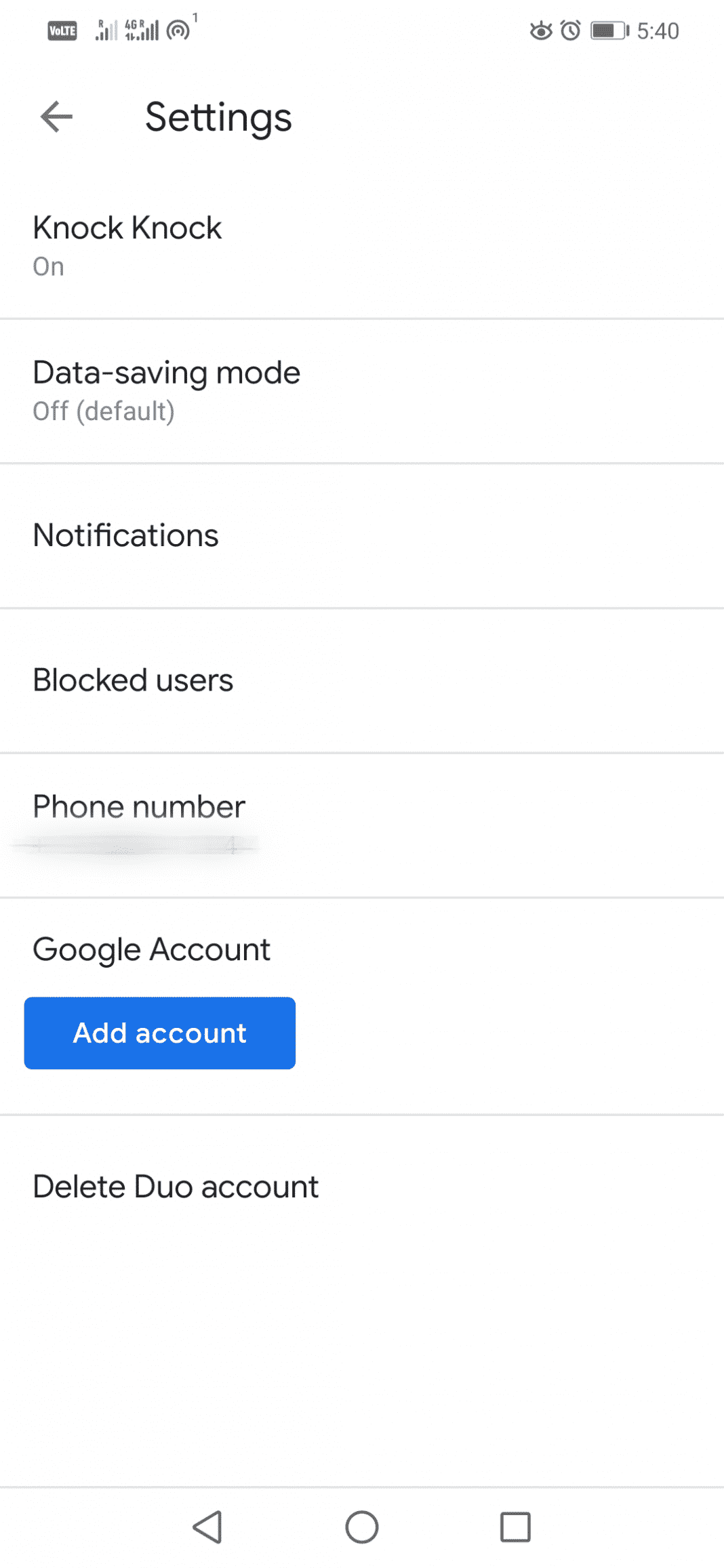The image displays a settings screen on a mobile device.

In the upper left corner, there is a gray icon featuring the text "V-O-L-T-E," accompanied by a 3 out of 5 data signal icon next to the letter "R," and a 5 out of 5 data signal icon next to the letter "V" or "4G". A Wi-Fi icon is also visible.

In the upper right corner, there's an eyeball icon, a clock displaying the time as 5:40, and a battery icon showing approximately 75% charge.

Below the top bar, a gray back arrow is positioned next to the word "Settings."

The main content includes various options:
- "Knock knock: On"
- "Data saving mode: Off (default)"
- "Notifications"
- "Blocked users"
- "Phone number" (the number itself is blurred out for privacy)

Additionally, there's a section labeled "Google account," featuring a blue button with the text "Add account" in white font. 

Beneath this, an option to "Delete Duo account" is listed. 

At the very bottom, standard navigation icons are present: a back arrow, a circle for the home screen, and a square for recent tabs.